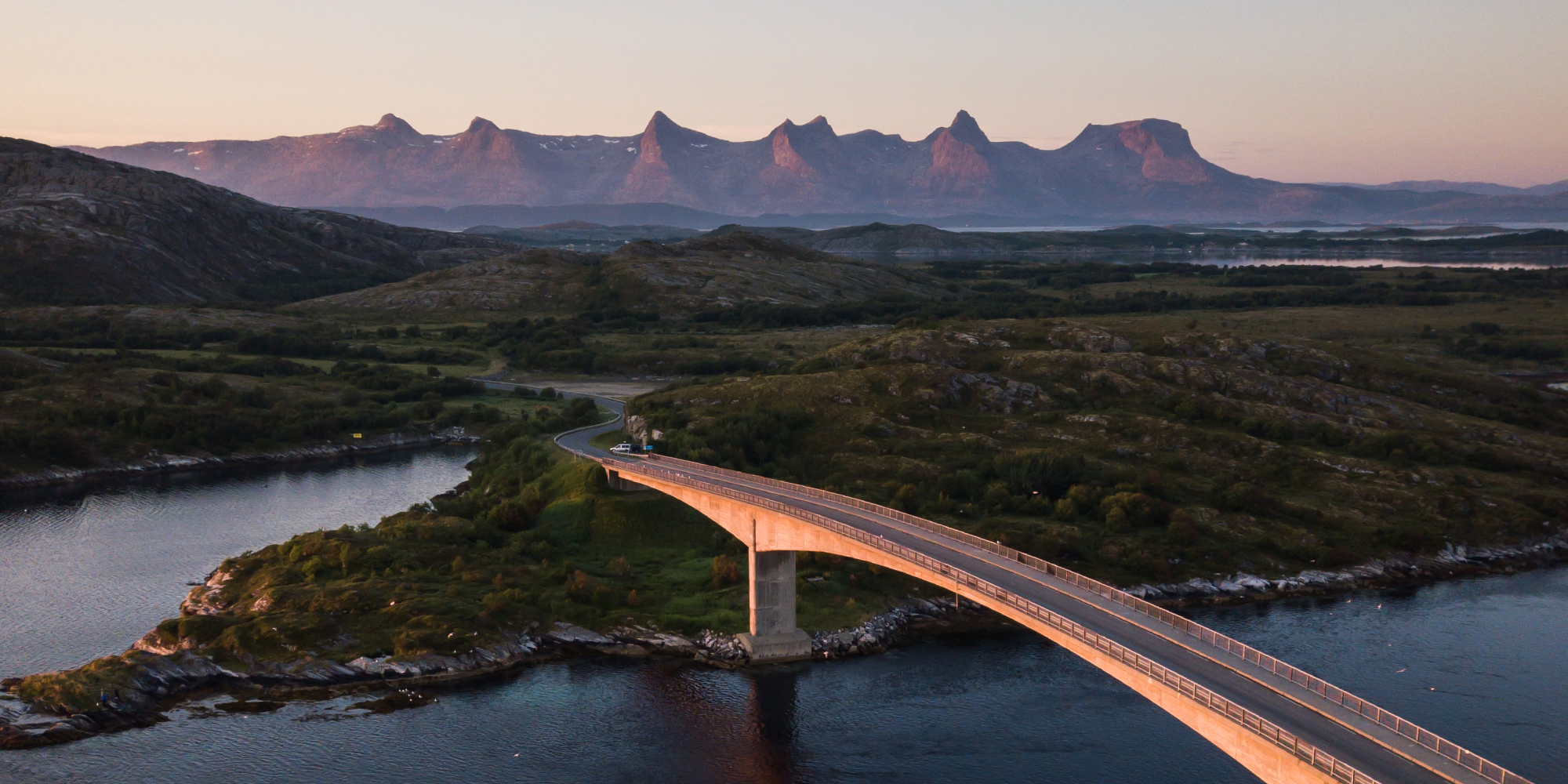A breathtaking aerial view captures a gracefully curved bridge spanning a deep blue river, set against the backdrop of a majestic mountain range under an overcast sky. The bridge, kissed by the sun, glows with warm orange hues along its sides while it winds through lush, dark green grassy hills dotted with gray stones at the water’s edge. Beyond the bridge, the river flows onward, with a meandering road stretching into the distance towards distant, reddish-tinged mountains, contrasting beautifully with the serene, natural landscape.